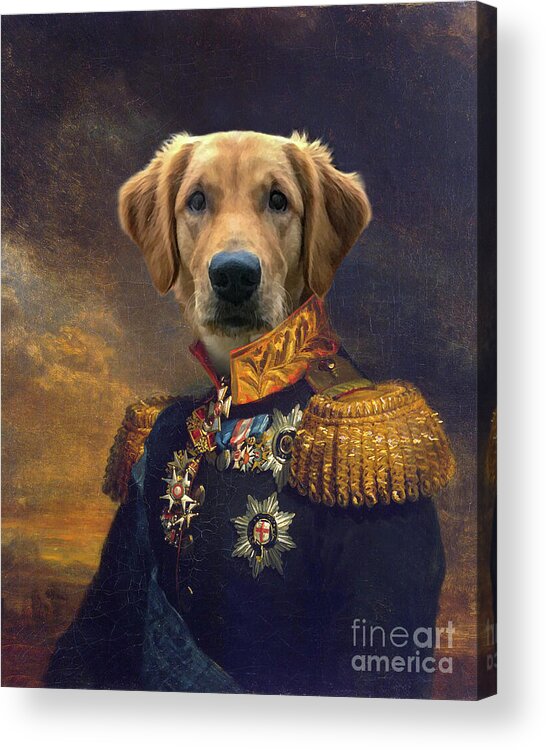The image depicts a highly detailed painting that merges fine art and surrealism. In the bottom right-hand corner, the words "fine art America" are inscribed in lowercase white font. The central figure of the painting is a golden retriever with lifelike, expressive eyes, which seems to have been superimposed onto the body of a human clad in an 18th or 19th-century military uniform. The uniform is richly decorated with numerous medals—some gold, silver, and adorned with blue and red ribbons—along with gold tassels on each shoulder and a large, elaborate gold collar. The background features a somewhat muted scene transitioning from dark, ominous clouds at the top to a subtle, subdued sunset near the bottom, creating a dramatic yet serene atmosphere. The golden retriever's face, staring directly at the viewer, adds a whimsical and thought-provoking contrast to the elaborate military attire.